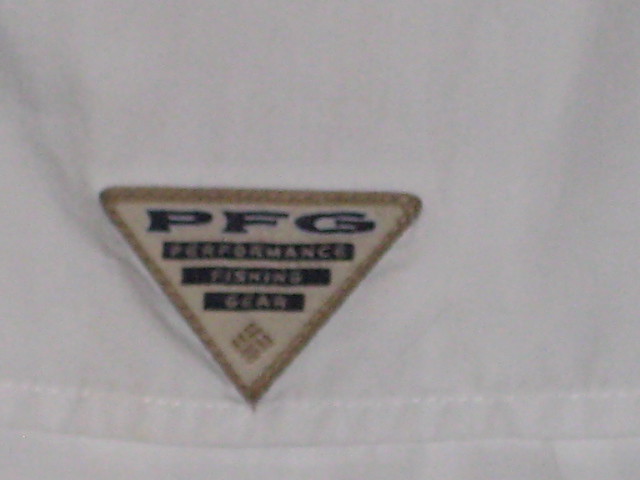This photograph is an extreme close-up of a label on a white fabric, likely from a piece of clothing. The image is slightly blurry, but the texture of the threads in the white fabric is visible. The object extends beyond the frame, but at its center, there is an upside-down triangular patch. This patch features a light brown border with white stitching. Inside the border, there is an off-white area containing the blue letters "PFG" in a large font at the top. Below it, three blue ribbons with white text read "Performance," "Fishing," and "Gear" in sequence. Additional stitching is visible near the bottom of the fabric, running horizontally. Despite the lack of clarity, the details of the patch and the intricate stitching make the nature of the label discernible.